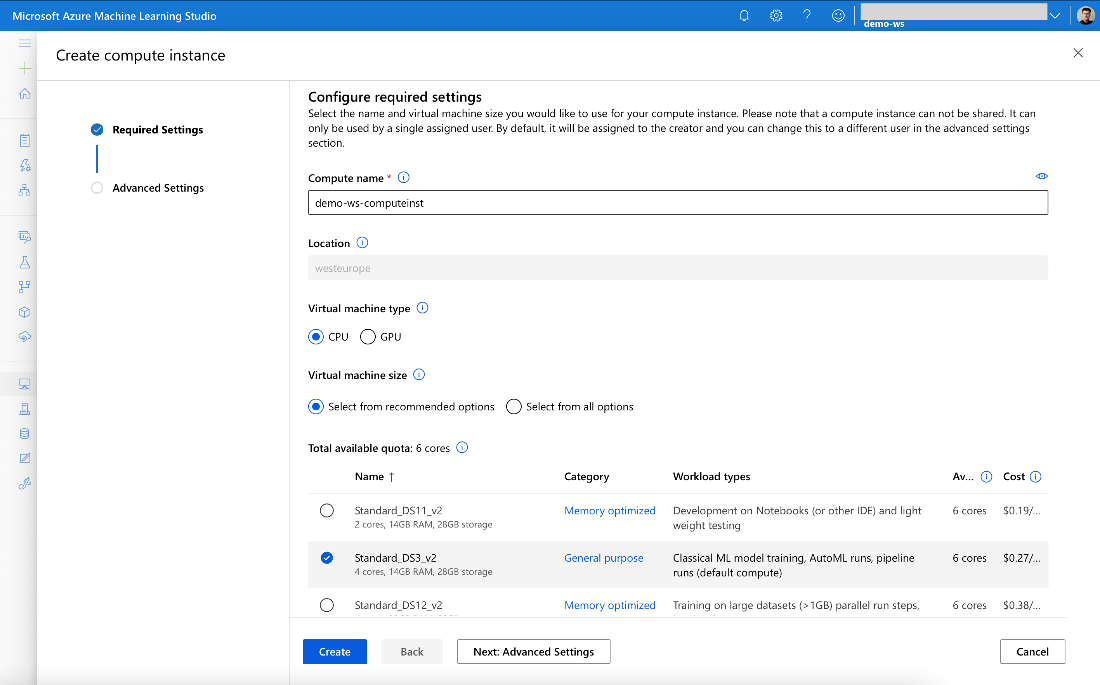The image captures a pop-up window on a computer screen within the Microsoft Azure Machine Learning Studio interface. The topmost area features a blue border with the title "Microsoft Azure Machine Learning Studio." Along the far right edge of the window, there is a gray section labeled "Demo."

At the center is a white pop-up screen titled "Create Compute Instance." On the left side of this screen, there is a section labeled "Required Settings," indicated by a check mark, and a blue line extends downward to a circle labeled "Advanced Settings." 

In the middle of the pop-up, under the heading "Configure Required Settings," there is an input bubble for "Compute Name," which has been filled in with "Demo WS Computerist." The section beneath shows the "Virtual Machine Type," where the "CPU" option has been selected. 

Further down, within the "Virtual Machine Size" category, the option "Select from Recommended Options" has been chosen. Following this, the "Standard DS3.v2" option is highlighted under "Total Available Quota."

At the bottom of the screen, the user has apparently clicked a blue button labeled "Create." Additionally, a button marked "Next: Advanced Settings" has been highlighted.